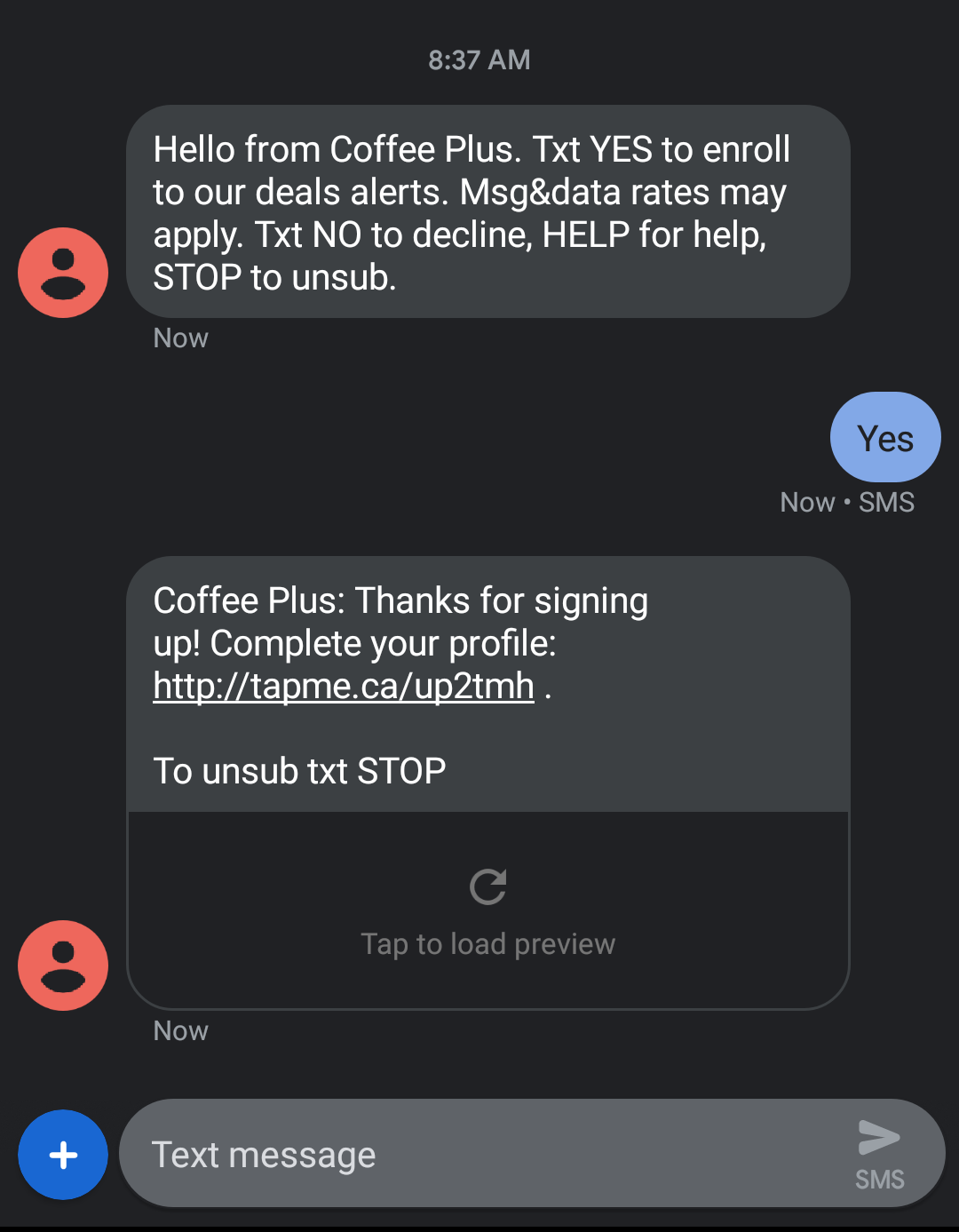The image is a cropped screenshot from a text messaging app set against a dark green background. It captures a conversation between a user and a service called "Coffee Plus." At the top, the time is displayed as 8:37 a.m. 

The first message, sent by "Coffee Plus," reads: 
> "Hello from Coffee Plus. Text YES to enroll in our deal alerts. Message and data rates may apply. Text NO to decline. HELP for help. STOP to unsubscribe."

Next to this message is a red circle icon with a black silhouette of a person, indicating the sender. Below it, marked with "Now," is the user's reply in a blue text bubble:
> "Yes"

Following this, "Coffee Plus" responds:
> "Thanks for signing up! Complete your profile" 

They include a link, below which it states:
> "To unsubscribe, text STOP."

There is a placeholder for an image or website preview that did not load, displaying "Tap to preview." At the bottom of the screen, there's a text input box labeled "Text message." To the right of this, a sending icon shaped like a paper airplane is shown, accompanied by an "SMS" label. On the left side of the text box is a blue circle with a white plus sign in the center.